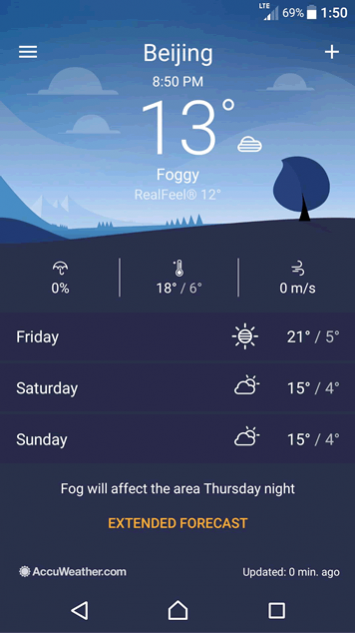This screenshot captures the home page of a mobile weather app. The background is a serene blue landscape featuring distant mountains and a solitary tree in the foreground to the right. Fluffy white clouds are scattered across the sky. 

At the top center of the screen, it displays "Beijing" with the current time marked as 8:50 PM. The temperature reads 13°F, while a subtext indicates fog with a real feel of 12°F. 

In the top right corner, the device time is noted as 1:50, with a battery level of 69% and an LTE signal status.

Directly below the main temperature readout, there's a horizontal row of additional weather details: 
- An umbrella icon with 0% precipitation chance,
- A temperature range showing 18°F / 6°F,
- A wind icon indicating calm conditions at 0 m/s.

Further down, a forecast list spans from Friday to Sunday, projecting temperatures of 21°F for Friday, 15°F for Saturday, and 15°F for Sunday. 

Below the forecast, a notice in text warns, "fog will affect the area Thursday night," followed by an orange-highlighted "EXTENDED FORECAST." The information is sourced from AccuWeather.com and was updated just moments ago.